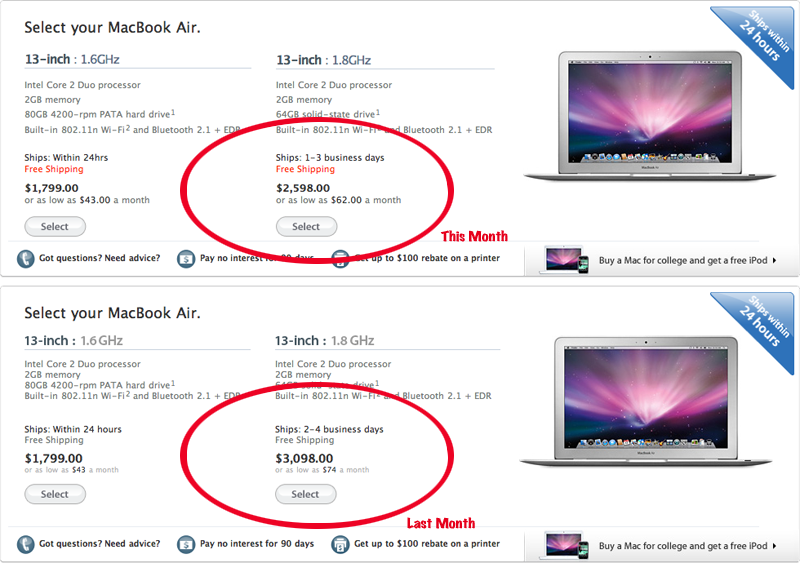A horizontal left-to-right image showcases a web page advertisement for selecting a MacBook Air. The web page is presented on a white background, giving it a clean and minimalist appearance. The advertisement is divided into two distinct sections, each outlined by a thin black border.

At the top left corner, bold black text reads, "Select Your MacBook Air, 13-inch, 1.6 GHz." Below this title, detailed specifications are listed, including the Intel Core 2 Duo processor, 2 GB of memory, and accompanying information about free shipping and pricing. Next to this section, a MacBook Air model is displayed with promotional details. The first option, priced at $2,598, is prominently circled with a red oval, drawing attention to it.

Beneath the top section, another similar MacBook Air advertisement is presented. This section again starts with the title, "Select Your MacBook Air, 13-inch," followed by specific details. The second model is listed at $1,799, while an upgraded option is highlighted with a red oval, showcasing a price of $3,098. Various icons and interactive elements are also present, indicating additional features or actions users can take, such as seeking advice or further information.

This neatly organized advertisement makes it easy for users to compare different MacBook Air models and their prices, visually emphasizing the highlighted options.